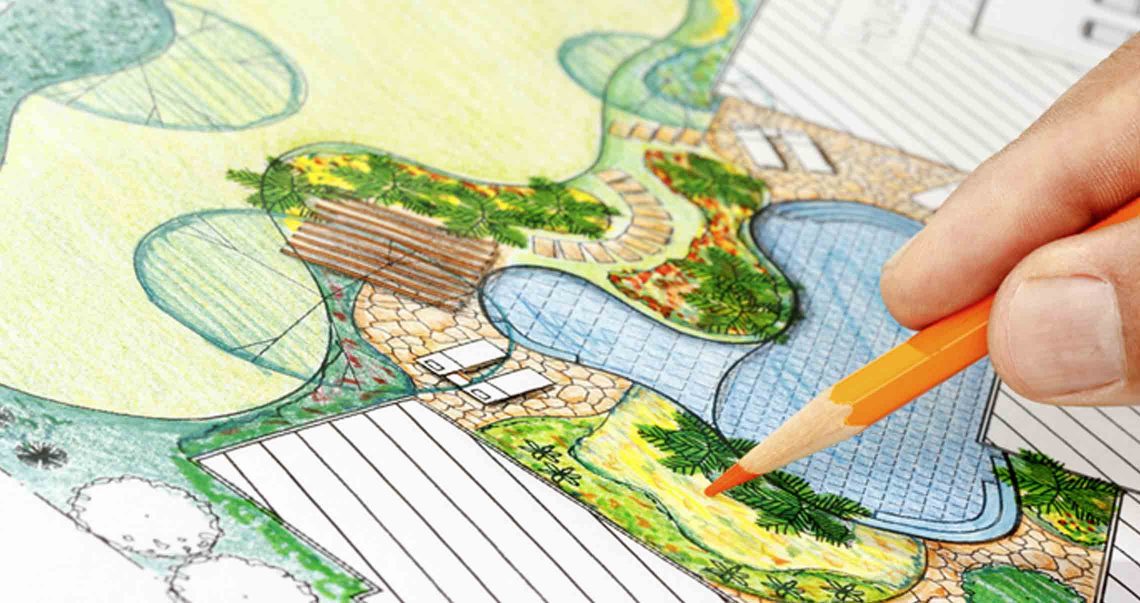In this detailed landscape-oriented photograph, a close-up shot captures the index finger and thumb of someone on the right holding a yellow colored pencil, actively sketching and coloring a sophisticated garden design. The primary focus of the drawing is a distinctive, large, peanut-shaped swimming pool complete with a long, curved extension on one side. Encircling the pool is a stone paver deck adorned with lounge chairs and a variety of tropical plants such as sago palms. 

In the background, we catch sight of the partially drawn and labeled house, albeit somewhat blurry and out of focus. Adjacent black and white outlines hint at additional structures, likely a deck or outbuilding, although these lack specific labels. The top left corner of the drawing reveals expanses of green, potentially symbolizing grass, interspersed with yellow areas possibly indicating sand. 

Noteworthy details include some yet-to-be-colored parts, like two large bushes in the bottom left corner, standing in contrast to the majority of the design that has already been vividly colored in varying shades of blue, green, and yellow. The presence of walkways and meticulously planned stone tiles accentuate the intricate and well-thought-out nature of this architectural landscape plan.